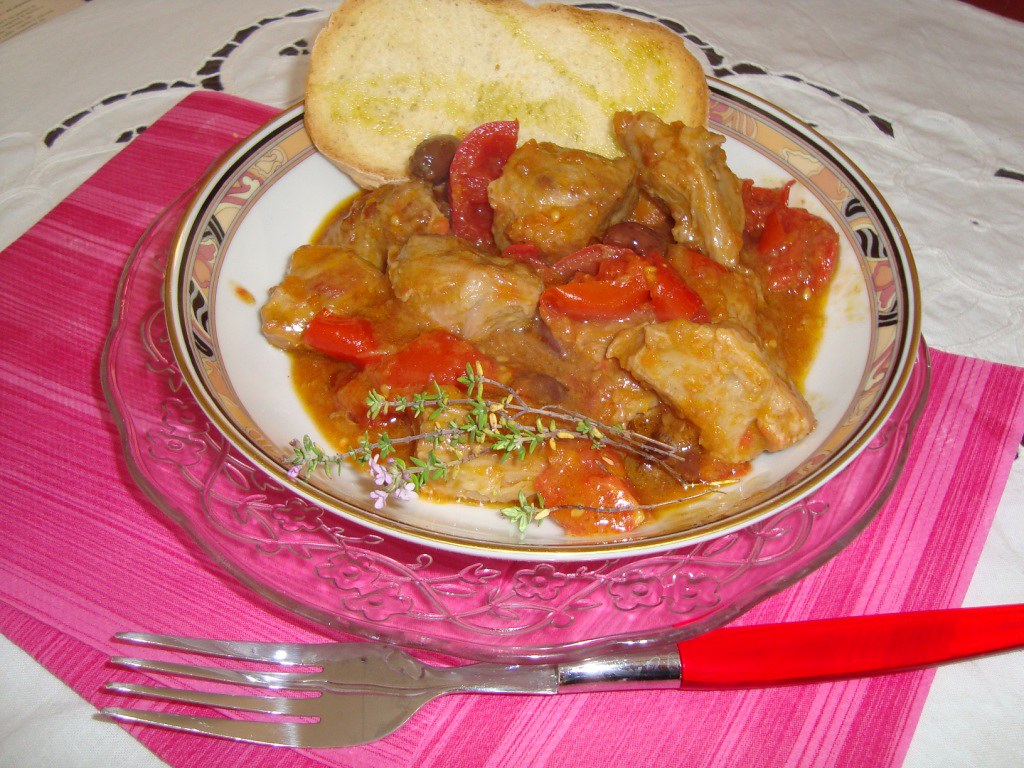In the image, a culinary presentation is displayed on a table. At the center, there is a shallow white bowl with a decorative edge featuring tan, black, and pink floral patterns. This bowl is placed on a clear glass plate adorned with a floral vine engraving. Inside the bowl, the main dish appears to be a chicken or pork entrée covered in a savory brown tomato sauce, studded with bits of red tomatoes and olives. Accompanying the dish is a slice of toast, possibly garlic or French bread, positioned prominently on the right side. A garnish featuring green herbs with small purple flowers, resembling rosemary, adds visual interest on the left side of the dish.

The glass plate sits atop a pink placemat, which is itself placed over a white doily tablecloth. A red-handled fork, with a chrome silver pronged end and potentially a plastic grip, lies beside the bowl to the left, completing the setting. The combination of textures and colors in the meal, along with the layered presentation of dishware on contrasting table linens, creates a visually appealing dining scene.